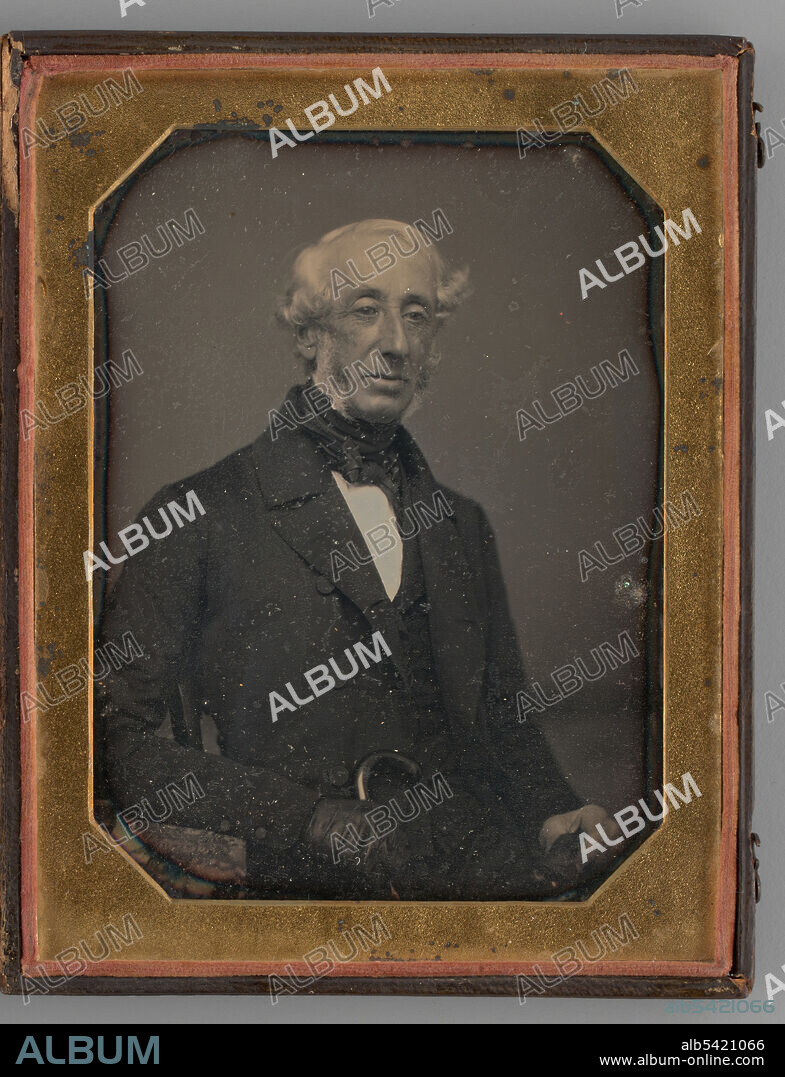This is a black and white photograph of an elderly gentleman, likely taken in the 1800s. The man, with his white hair and prominent sideburns but no beard or mustache, has a somber expression and slightly tilts his face toward the bottom right of the image. He is dressed in black attire, including a suit jacket, vest, and a scarf or cravat around his neck, with a white shirt visible underneath. The image is encased in an old, distressed wooden frame with a brown panel that appears dirty and cut up in some areas, contrasting against a gray background. Surrounding the photo, a gray-bordered octagonal shape, with varying side lengths, encloses the man's portrait. Watermarks of the word "ALBUM" in both solid and hollow white letters are diagonally spread across the image. At the bottom, "ALBUM" is prominently displayed in a black bar, accompanied by the identifier "ALB5421066" and the URL "www.album-online.com."